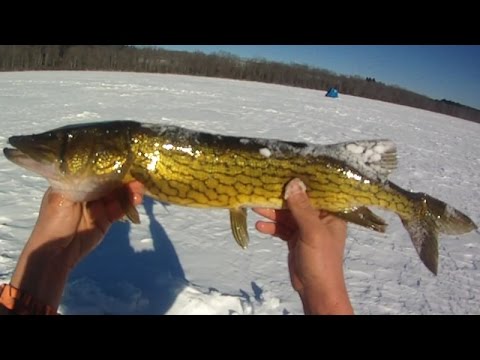This image captures a low-resolution, first-person perspective of a man holding a freshly caught fish in both hands after an ice fishing expedition. The photograph, framed horizontally with black bars at the top and bottom, showcases the man’s shadow partially obscuring his left hand and the snowy ground beneath. The fish, held prominently, has a striking appearance with shiny, reflective scales that transition from a dark brown spine to a golden-yellow body, accented with brown vein-like markings. Snow dusts the top back fin and other parts of the fish. The setting is a clear, sunny winter day by a frozen lake, blanketed in pristine white snow. In the distant background, a blue ice fishing hut and a line of leafless brown trees are visible against a vibrant blue sky, devoid of clouds.